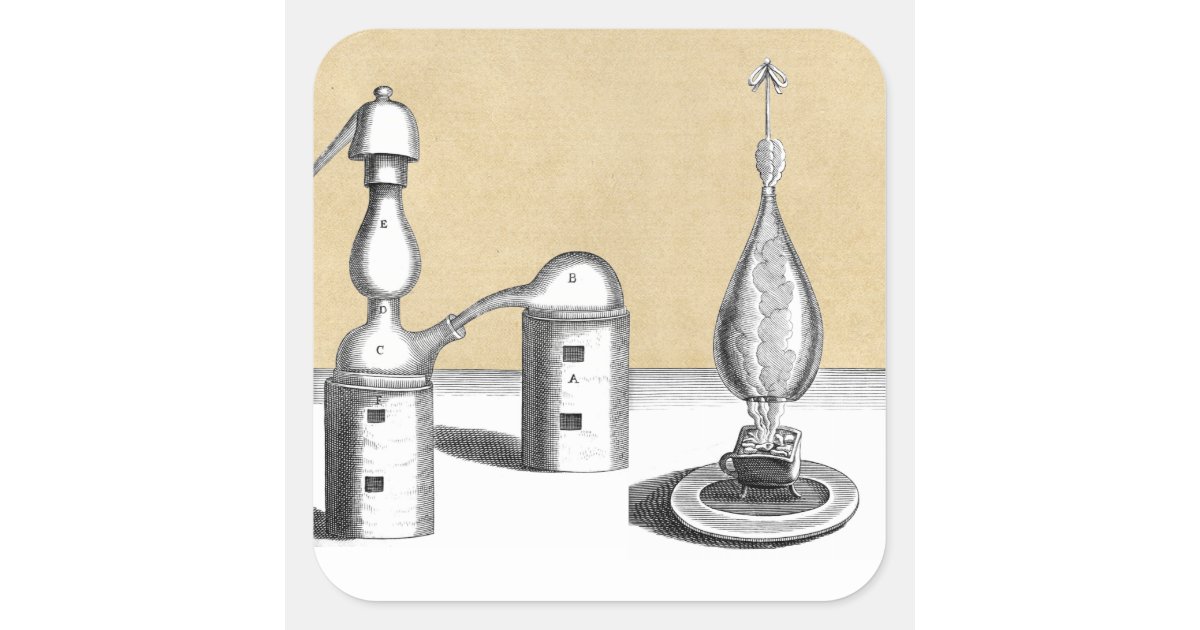The illustration appears to depict an assortment of alchemical or chemistry equipment meticulously drawn in grayscale, set against a light beige background with a white surface beneath them. Central to the image is a complex assembly of tube-like and cylindrical shapes with intricate labels. On the left, a prominent sequence starts with a cylinder labeled F, which supports a bulbous item marked D and C. This is crowned by a dome-shaped piece labeled E. A spout from this middle section connects to another bulbous item labeled B, positioned on a cylinder marked A. To the right, a separate element shows what resembles a Bunsen burner with an active flame, surmounted by a glass container that narrows toward the top, capped with a glass lid. Each piece has detailed black ink lines, contributing to a heavy, slightly chaotic feel, with labels ranging from A to E correctly but missing the sequential label D, suggesting some complexity or intentional omission in the illustration.